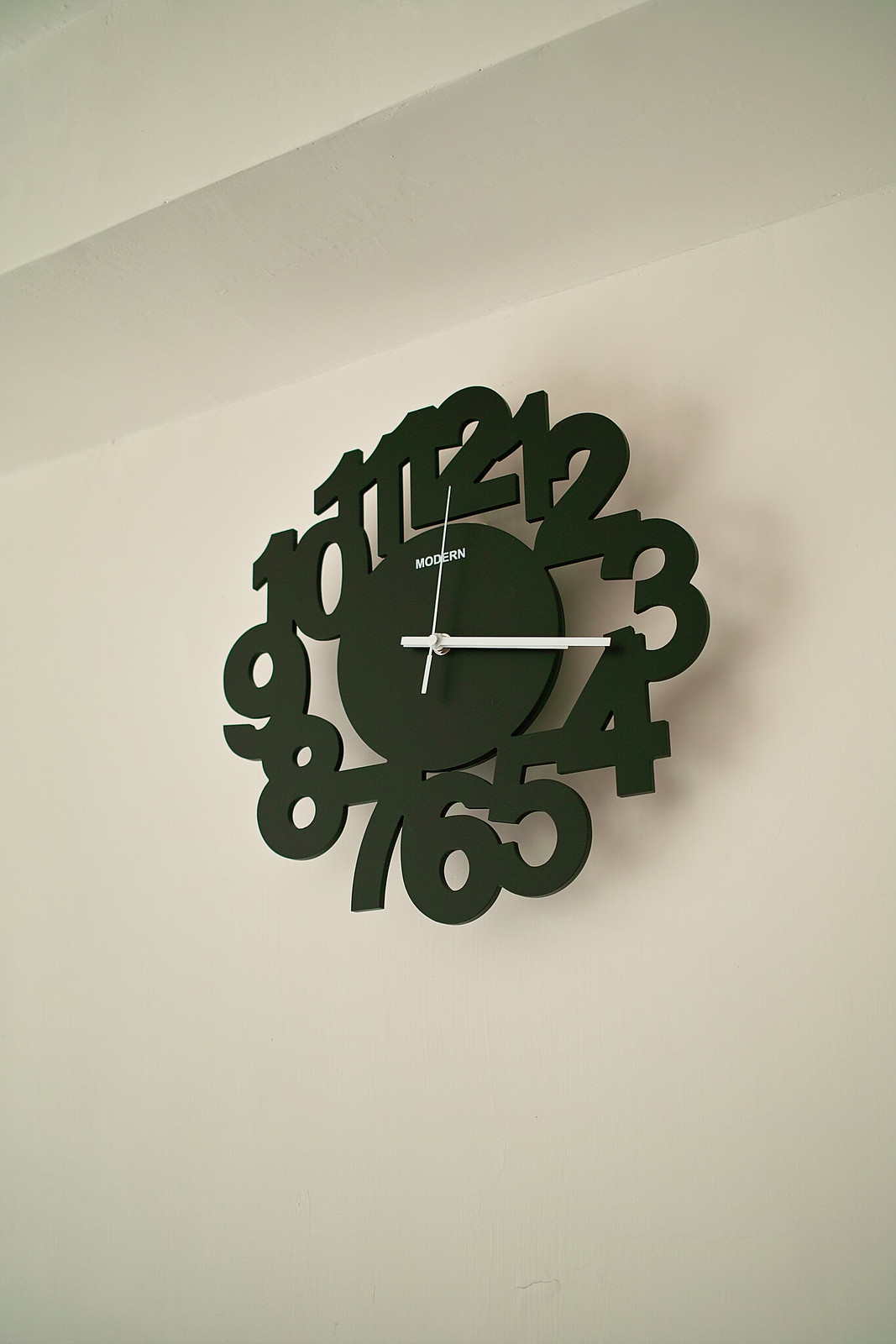The image depicts a green clock hanging on an off-white wall. The clock lacks a traditional frame; instead, its design features standalone numbers from 1 to 12 creating the outline. These numbers are closely positioned and partly interconnected, with certain numbers directly attached to a central green circle. In the center, the clock bears the word "modern" in small white text. The clock's hour, minute, and second hands are also white, contrasting against the green. The hands are indicating a time around 3:16, with the second hand precisely at 12.